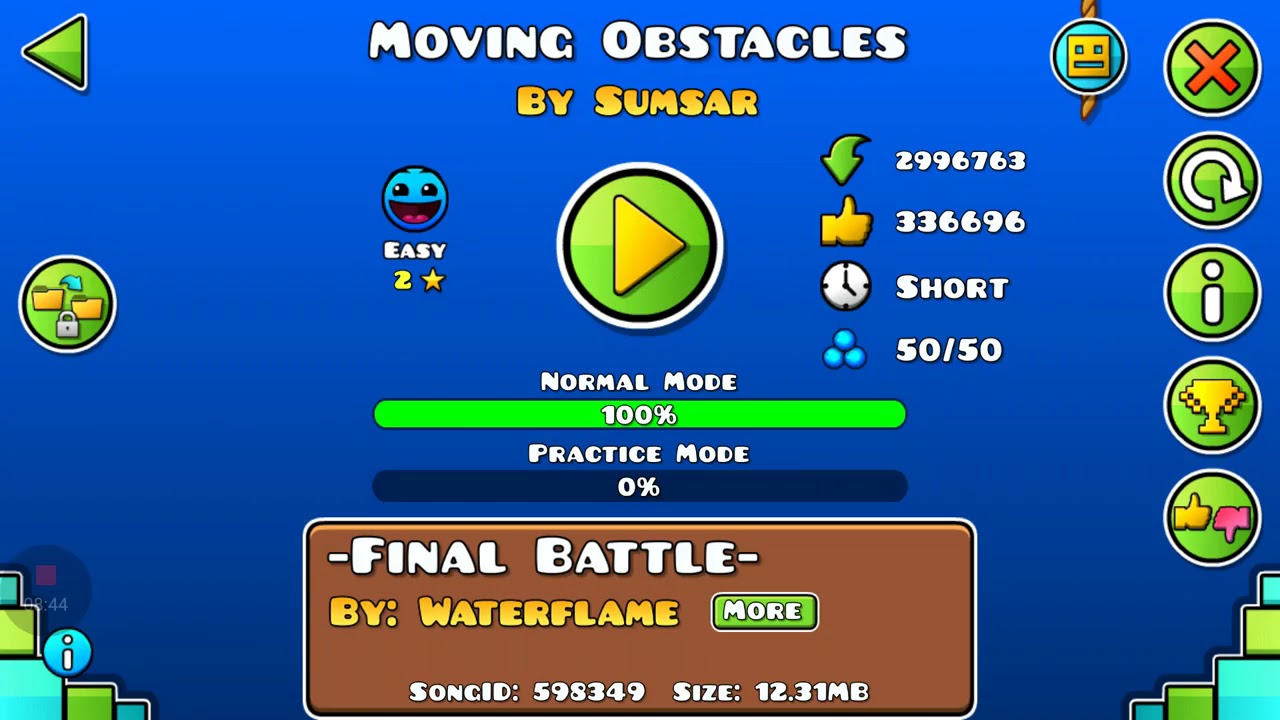The image is a brightly colored home screen of a digital game titled "Moving Obstacles" by Samsar. Dominating the background is a bold blue color. At the very top, the game title is in large, clear text with "by Samsar" written in yellow beneath it. Central to the screen is a large green circular play button featuring a yellow triangle. Adjacent to the play button, on the left, is a blue smiley face with "Easy" labeled beside it.

Below the play button, there's a sequence of labeled modes. "Normal mode" is shown with a green bar indicating 100% completion, followed by "Practice mode" with 0% completion. At the bottom of the screen, a brown box prominently features "Final Battle" in white text with "by Waterflame" written in yellow. Next to it, another green box with white text says "More." Below these boxes, "Song ID: 598349" and "Size: 12.31 MB" are detailed.

The top-right corner of the screen houses various interactive icons including an X, a reverse arrow, an information button, a trophy, thumbs-up, and thumbs-down. The buttons are highlighted in vibrant colors such as lime green, yellow, red, white, and pink. In the bottom corners, smaller boxes provide additional options in light aqua blue and light green tones. The arrangement and diverse color palette give the screen an engaging and lively appearance, enhancing the gaming experience reminiscent of classic games like Mario and Flappy Birds.